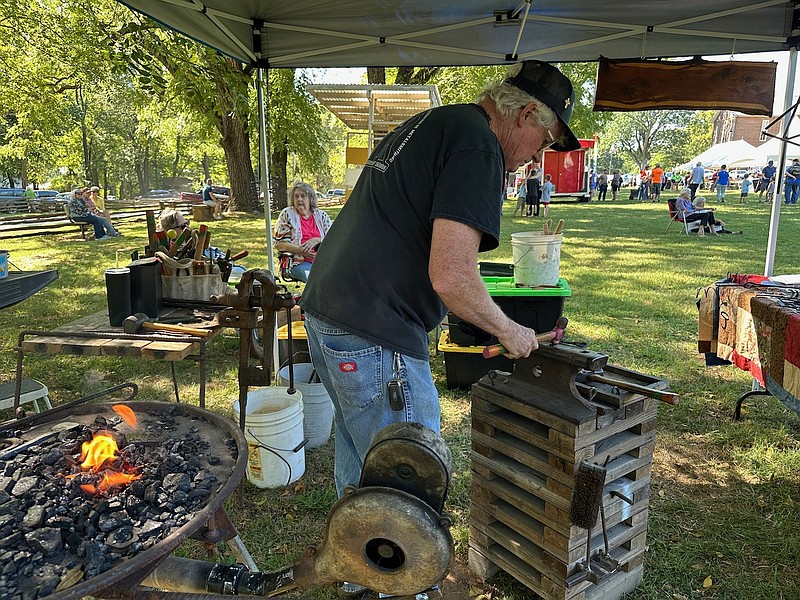In this vibrant outdoor scene at a public event, likely a fair in a recreational park, we see a blacksmith engrossed in his craft under the shade of a tent. The man, appearing to be in his 60s or 70s, is clad in blue jeans, a short-sleeved black shirt, a black baseball cap, and a cardbinder with keys clipped to a belt loop. Leaning intently over a small black anvil set on a stack of brown wooden planks, he hammers a piece of metal with a ball-peen hammer. To his right, a wooden table is laid out with various tools, including a small hammer and a black cup with a straw. In the bottom left corner, a metal barbecue grill glows with burning charcoal. Behind him, to the left, one can spot a couple of five-gallon white buckets, one filled with water. The backdrop features lush green grass, a few trees, a road, and a fence, suggesting a serene yet bustling environment. Among spectators, a woman with gray hair wearing a pink shirt and a white cover is seated, adding to the communal ambiance of the park event.